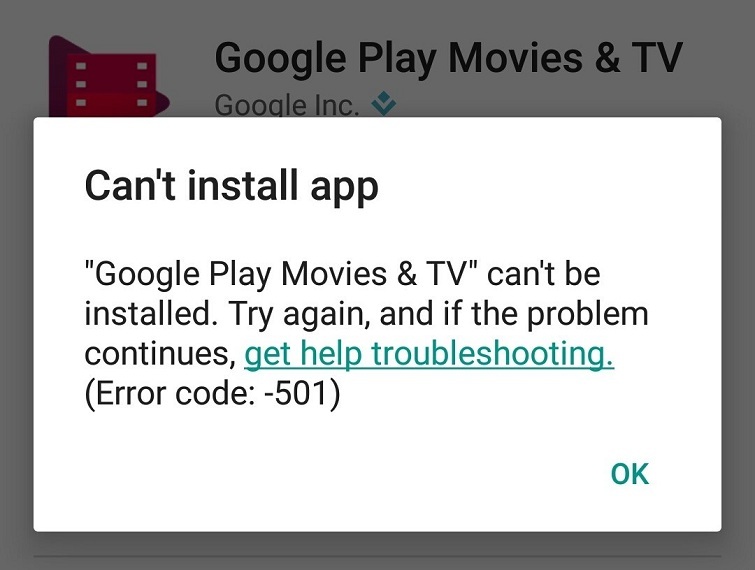The image displays the Google Play Store interface, featuring an error message pertaining to the installation of the "Google Play Movies & TV" app. The primary background of the error section is white, while the text is predominantly in black. The specific error message states, "Can't install app 'Google Play Movies & TV.' Try again, and if the problem continues, get troubleshooting. Error code: -501.” The phrase "get troubleshooting" is highlighted in green, as is the "OK" button located at the bottom right corner of the error message.

At the top of the error message, the app's details are displayed. In the center, "Google Play Movies & TV" is written in black. To the left of this text, there is the app’s icon, which features a stylized play button. The play button is depicted as a maroon triangle facing right, integrated into a square that has a slightly red tint, reminiscent of a video camera or film motif, collectively forming the recognizable Google Play Movies & TV logo. The overall interface follows the clean and minimalist design typical of Google’s aesthetic.